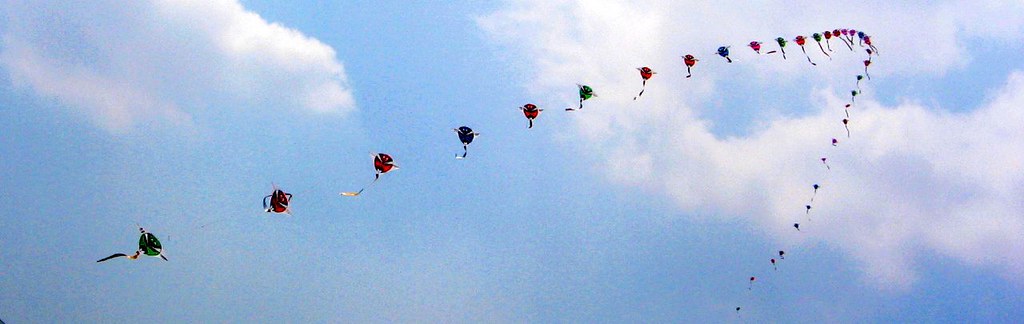The image is a vibrant color photograph with a panoramic, long rectangle orientation, featuring a bright blue sky adorned with fluffy white clouds. Dominating the scene is a striking V-shaped formation created by a continuous line of kites, intricately strung together. This formation starts from the bottom left of the photo, ascends toward the top right, and then gracefully loops down, forming an elegant curve. There are approximately 40 kites in total, with about 20 kites along each arm of the V-shape.

Each kite in this impressive display is similarly designed, with a circular shape featuring three prongs extending outward and a streamer-like tail trailing behind. The kites boast a variety of colors, alternating between green, red, blue, and more, adding a vibrant spectrum to the composition. Every individual kite appears as if it were a face, with a solid background color and striped patterns resembling eyes. This captivating display creates a dynamic and picturesque scene against the serene backdrop of the sky.